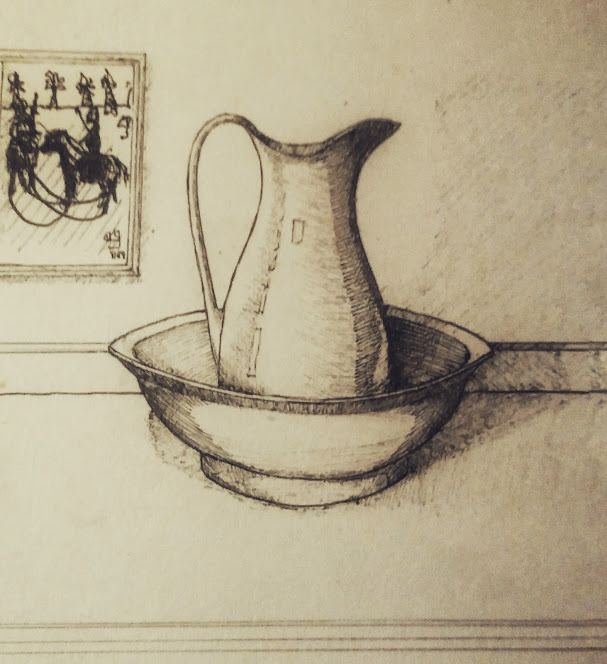This detailed hand-drawn image features a prominently large mug, placed within a substantial bowl. The mug, which is possibly intended to be metal, is designed for pouring either milk or water, indicated by its significant size and the curved rim suited for pouring. The shading work is particularly commendable, with a range of tones achieved using a single pencil, accentuating depth and dimension through meticulously applied shadows. In the background, a framed painting is visible on the wall. This painting depicts a scene with several soldiers on horseback, further enriching the overall composition and narrative of the drawing.